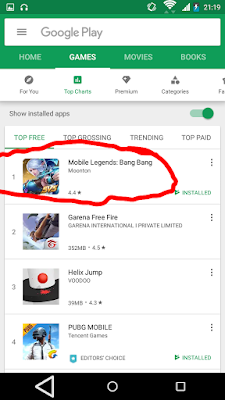Screenshot of a Google Play Store screen on a smartphone, focusing on the "Top Charts" tab within the "Games" section. At the top of the screen is a green banner containing a white search bar labeled "Google Play." Below the banner, various sections are listed: Home, Games (selected), Movies, Books, For You, Top Charts (selected), Premium, Categories, and Show Installed Apps (slider button set to on). The displayed chart categories include Top Free (selected), Top Grossing, Trending, and Top Paid.

Ranked first, "Mobile Legends: Bang Bang" has been marked with a red circle and is installed on the device. The game features an icon of a busty young woman with silver hair. In second place is "Garena Free Fire" by Garena International Private Limited, sized at 352MB and rated 4.5 stars. Third-ranked "Helix Jump" by Voodoo is 39MB in size and has a rating of 4.3 stars. Coming in fourth is "PUBG Mobile" by Tencent Games, designated as an Editor's Choice and listed as installed. Its icon depicts a person dressed in a white collared shirt with a black necktie, wearing a steel gray helmet, and an assault rifle strapped to their back. This PUBG Mobile icon is notably taller than it is wide.